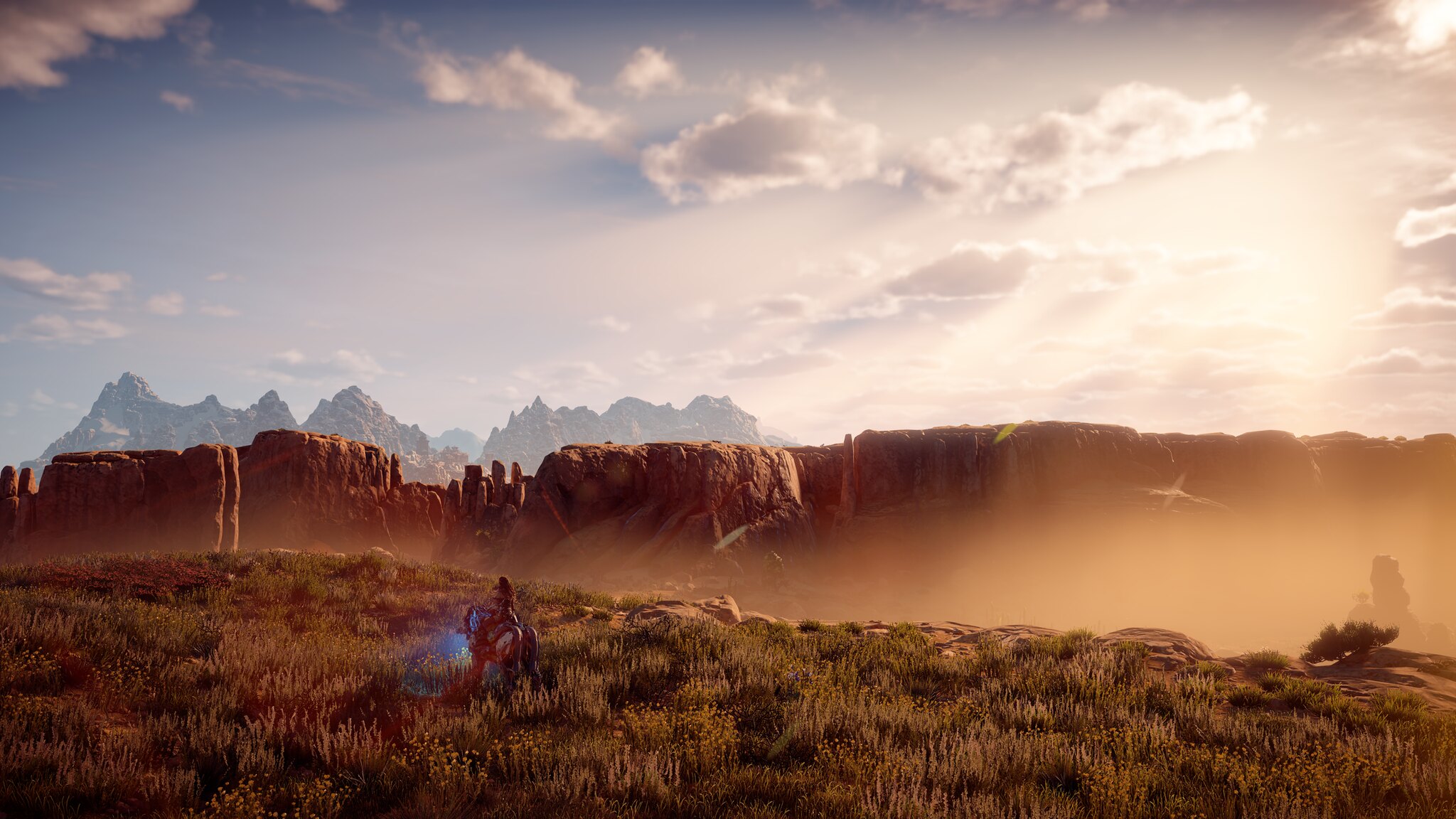The image is a highly detailed and realistic scene that evokes the aesthetic of a video game, yet could also be mistaken for a photograph or painting. Set in a rugged, desert-like environment, the foreground features a vast expanse of green and brown grass. Central to the scene is a canyon with steep, brown cliffs and rock formations that dominate the landscape, creating a dramatic crevice that splits the terrain. On the bottom left, a character dressed in orange and crouching—possibly a cowboy—is visible, holding a device emitting a blue light. In the distance, immense rocky formations and rugged mountain ranges reminiscent of the Grand Tetons rise, their peaks free of snow and bathed in sunlight. The sky above is a vivid blue, filled with fluffy clouds, and the overall lighting suggests a warm, golden hour ambiance with the sun positioned low on the right, hidden behind the clouds but intensely illuminating the scene. This atmospheric lighting casts an orange hue across the landscape, enhancing the realism and beauty of this wild, Western vista.